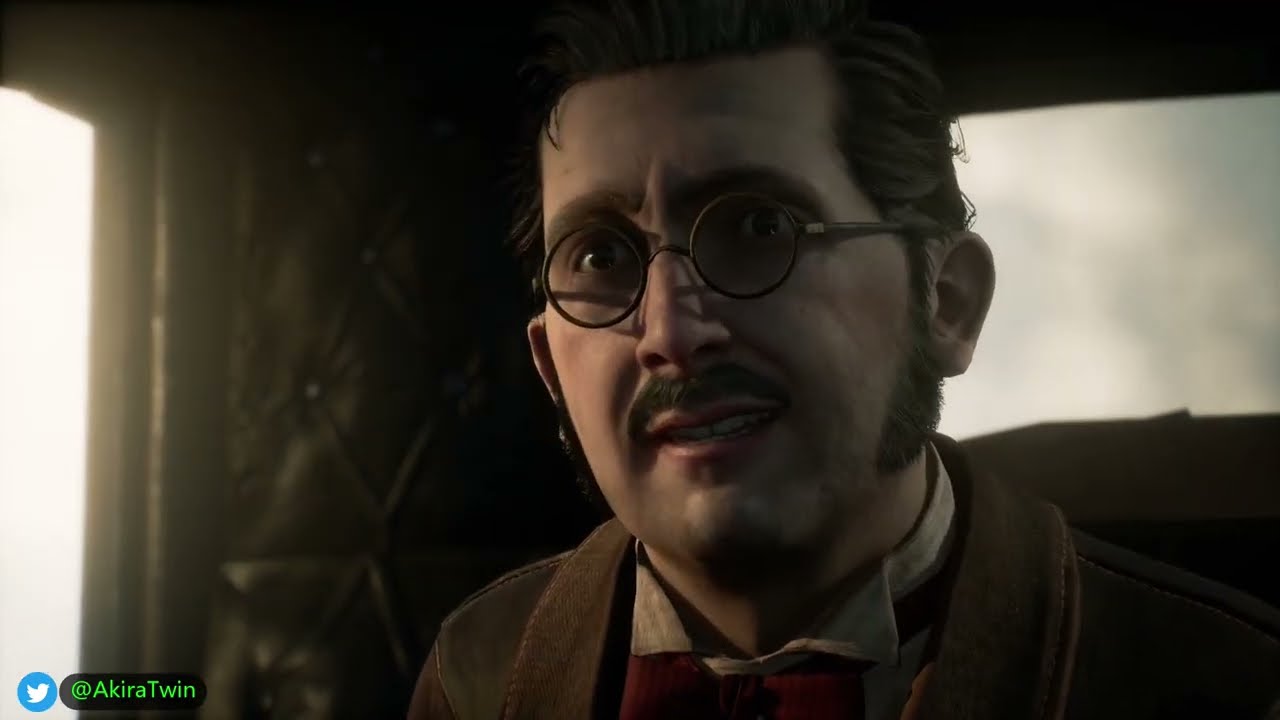The image captures a detailed 3D-rendered scene, possibly a screen capture from a video game or a rendered movie. A man is seated in what appears to be the back of a carriage or an old-fashioned vehicle, characterized by its dark black leather interior with padded surfaces. The scene is illuminated by natural light coming through an open window to the left and another window behind him on the right, revealing a gray sky outside. The man has fair, but slightly darkish Caucasian skin with swept-back black hair, thick sideburns that extend halfway down his cheeks, and a prominent black mustache. He wears round wire-rimmed glasses and has a serious, yet not unhappy expression, possibly conveying concern or confusion. His attire consists of a brown suit jacket, a red sweater, and a white shirt with a pointed collar, complemented by a red bow tie. In the bottom left corner of the image, a Twitter logo is visible, accompanied by the username "@AkiraTwin" in green text, suggesting that this image might be part of an internet stream or a shared social media post.